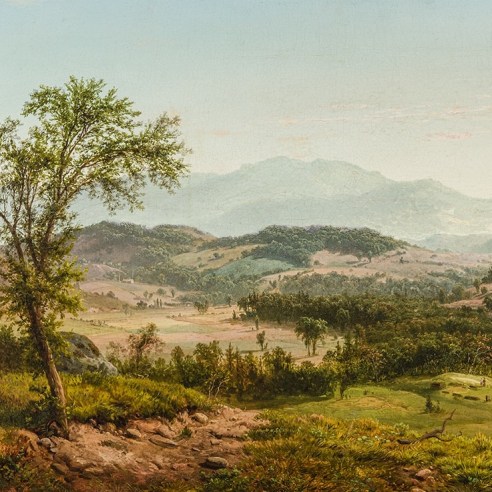The image portrays a serene landscape, likely an older photograph or painting, with a slightly faded appearance. The top of the image features a blue-gray sky with wispy, thin clouds, gradually transitioning to a lighter blue-gray hue. Distant hills, shrouded in a foggy gray, rise in the background, creating a tranquil backdrop. 

In the near foreground, a prominent tree occupies the left side, its trunk emerging from a patch of round dirt that descends down the hill. This tree leans slightly to the left, with branches arching upward and toward the right, adorned with vibrant light green and yellowish-green leaves. Surrounding the tree are scattered rocks and greenery. 

The right side of the foreground is verdant, with patches of green land and bushes suggesting a tended area, perhaps a former water area now dried out. A curvy row of green plant trees delineates the land from the section behind, which resembles a patchwork of farming fields in green and brown hues. The midground features rolling green hills dotted with clusters of vibrant green treetops while a few additional trees populate the center-right. There is no visible sign of human or animal presence, lending to the overall quiet and untouched nature of the scene.